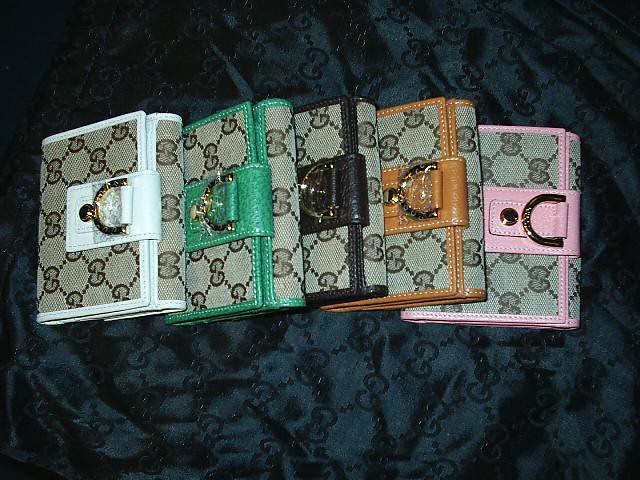This image features a collection of five foldable Gucci wallets, distinguished by their iconic pattern and design. Each wallet exhibits a unique border color while sharing a consistent tan-beige Gucci emblem pattern. The border hues are as follows, from left to right: white, green, black, camel khaki, and baby pink. These wallets are equipped with gold hardware, some pieces of which are still protected by plastic wrappings, implying they might be part of a new collection or a seller's display. The wallets rest on a navy blue blanket, also monogrammed with the Gucci logo, enhancing the brand's luxurious presentation.